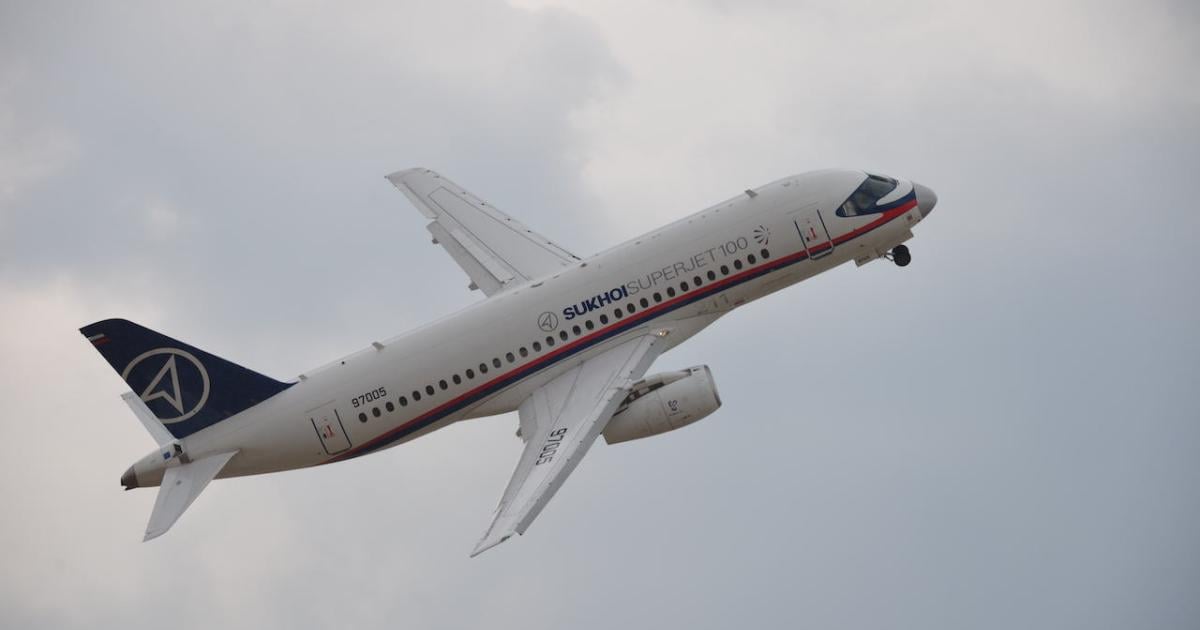This detailed color photograph captures a Sukhoi Superjet 100 airliner climbing against a gray, cloudy sky. The aircraft is depicted with its nose up, tail to the left, and nose to the right, indicating it is ascending. The fuselage predominantly showcases a white exterior adorned with a blue and red stripe that stretches from the tail to the nose, passing above a line of passenger windows. Elegantly inscribed in blue text near the front of the plane is the word "Sukhoi," followed by "Superjet 100" in light gray text. The tail number "97005" is prominently displayed towards the rear of the fuselage. The vertical stabilizer, or tail fin, boasts a blue background featuring a distinctive logo: an arrow pointing upwards encircled in white. One engine is visibly mounted under the nearest wing. The airliner's overall design, with two additional white pieces accentuating the blue tail, is set against the dramatic backdrop of the overcast sky, adding a sense of dynamic motion to the scene.